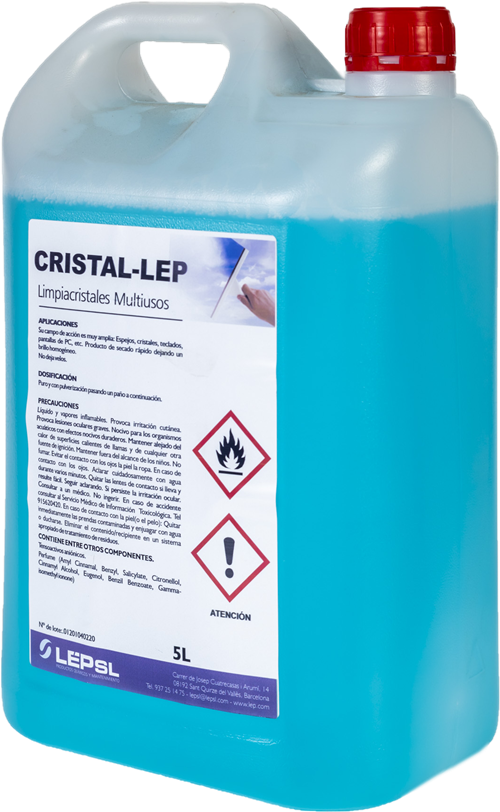The image features a large plastic jug of blue cleaning solution set against a white background. The jug is approximately a foot tall and has a semi-transparent, vertical rectangular shape, allowing the turquoise liquid inside to be partially visible. It is about 80-90% full, leaving some empty space at the top. The jug is equipped with a left-hand side handle for easy gripping and a circular spout on the right-hand side sealed with a red cap.

The front of the jug is adorned with a white, rectangular label. At the top of the label, "CRISTALLEP" is prominently displayed in black letters. Below this heading, there are instructions and details written in Spanish, including the phrases "Limpia Cristales Multiusos," which translates to multipurpose glass cleaner, as well as information about the product's application, dosage, and precautions. The label also features caution icons, such as a red diamond with an exclamation point and another indicating flammability hazards. At the bottom of the label, the letters "LPSL" are printed.